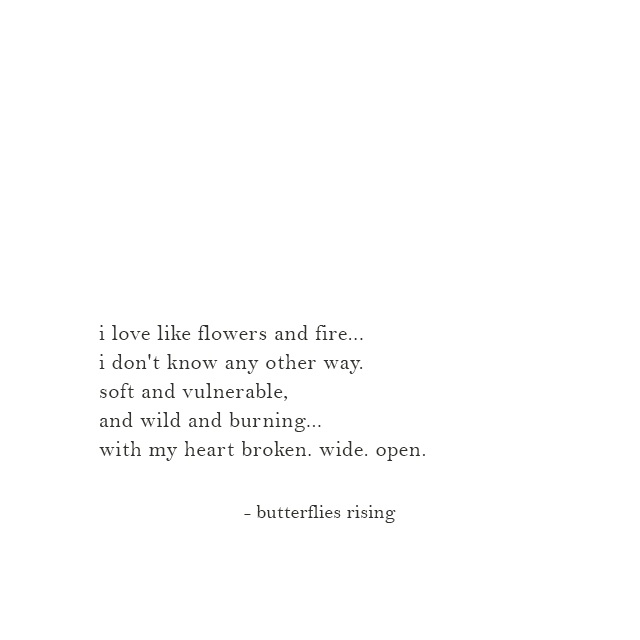The image is a simple, minimalist composition featuring black text on a white background. The text, all in lowercase letters and left-justified, appears to be a poem or quote spanning five lines. It reads:

"i love like flowers and fire,  
i don't know any other way.  
soft and vulnerable,  
and wild and burning,  
with my heart broken. wide. open."

The text is possibly rendered in Garamond font and the punctuation includes an ellipsis and periods for stylistic emphasis. Below the poem, attributed in lowercase black letters, is the name "butterflies rising" preceded by a dash, indicating the author. The overall aesthetic is one of simplicity and emotional intensity, conveyed through the poetic structure and the stark contrast of black text on a white background.